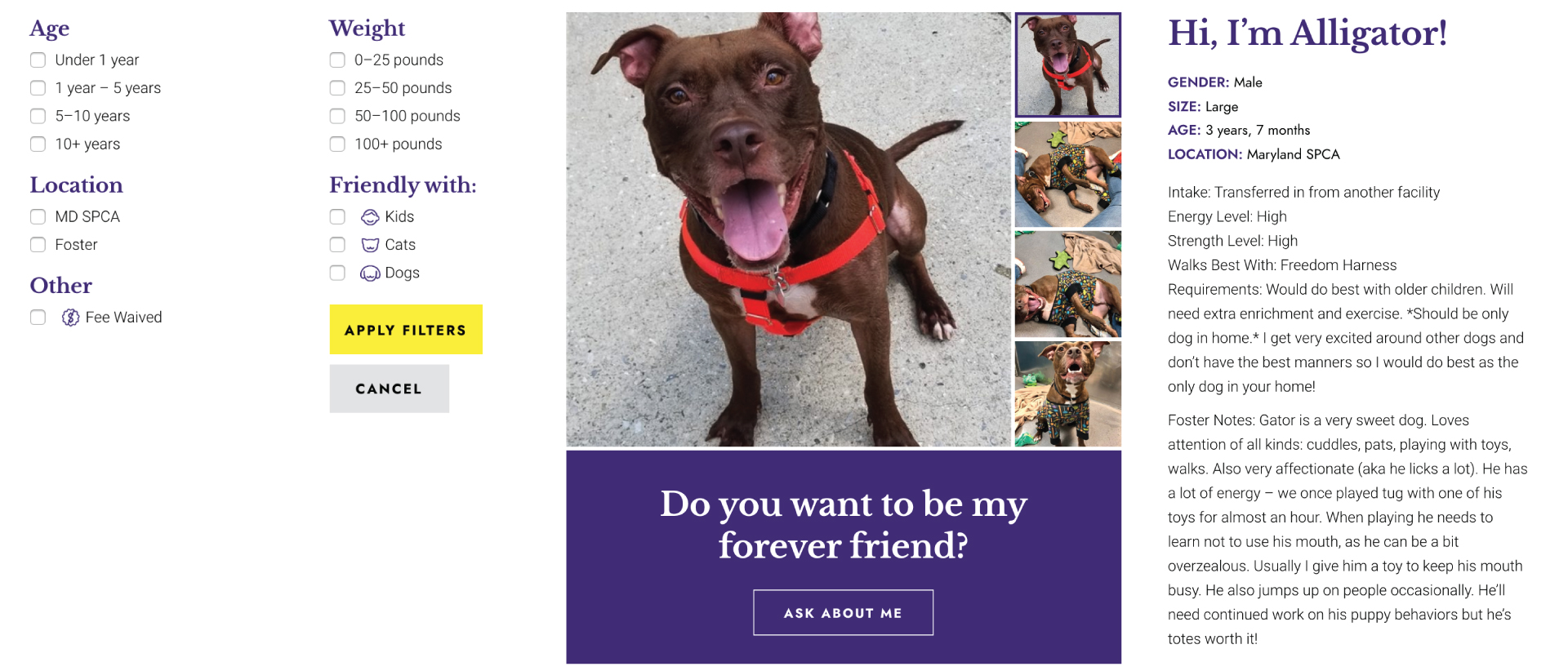This is a detailed screenshot from a pet adoption website. The layout features three columns of information. On the left column, several filtering categories are presented with purple text headers. The first category, "Age," includes four checkboxes for age ranges: under one year, one to five years, five to ten years, and ten plus years. The next section is "Location," listing checkboxes for "MDSPCA," "Foster," and "Other." An additional checkbox with a purple dollar sign icon indicates a "Fee Waived" option. 

Moving to the next column, categories begin with "Weight," offering four checkboxes for weight ranges: 0 to 25 pounds, 25 to 50 pounds, 50 to 100 pounds, and over 100 pounds. This is followed by the "Friendly With" section, accompanied by three checkboxes labeled "Kids," "Cats," and "Dogs." Below these filters are two buttons: a yellow "Apply Filters" button and a gray "Cancel" button.

The central section of the screenshot shows a vibrant picture of a dog. The dog, colored purple with a red harness and black collar, is captured sitting and looking up at the camera. To the right of this main image are four smaller pictures depicting dogs in various outfits and poses, both seated and lying down. Beneath the main dog image, a purple box states, "Do you want to be my forever friend? Ask about me."

On the right column, the information is presented in purple text, introducing the dog as "Hi, I'm Alligator." The specifics listed include gender (male), size (large), age (three years and seven months), and location (Maryland SPCA). Two paragraphs of small text follow this introductory information.